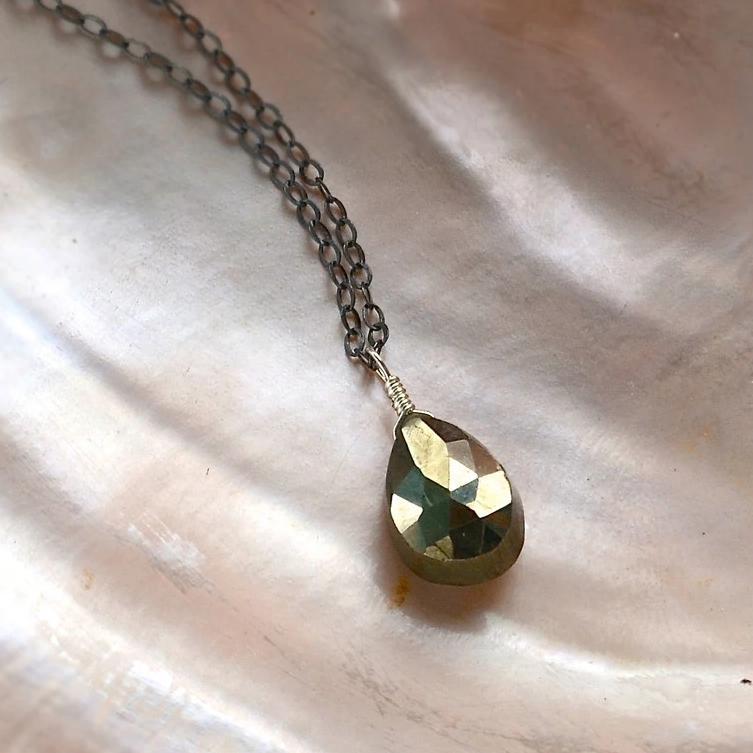In the photograph, a delicate necklace with a small-link chain takes center stage, draped elegantly in what appears to be an iridescent, clamshell-like background. The chain exhibits a subtle gray hue, comprised of tiny oval links that add a refined texture to the piece. Suspended from the chain is a striking teardrop-shaped pendant, its surface a glossy interplay of gold and black with hints of white shimmering under the light. The pendant's facets create a captivating array of reflections, accentuating its elegant design. The image itself is a vertical rectangle, slightly taller than wide, amplifying the vertical grace of the necklace against the contrasting darker grays in the upper right corner of the background.